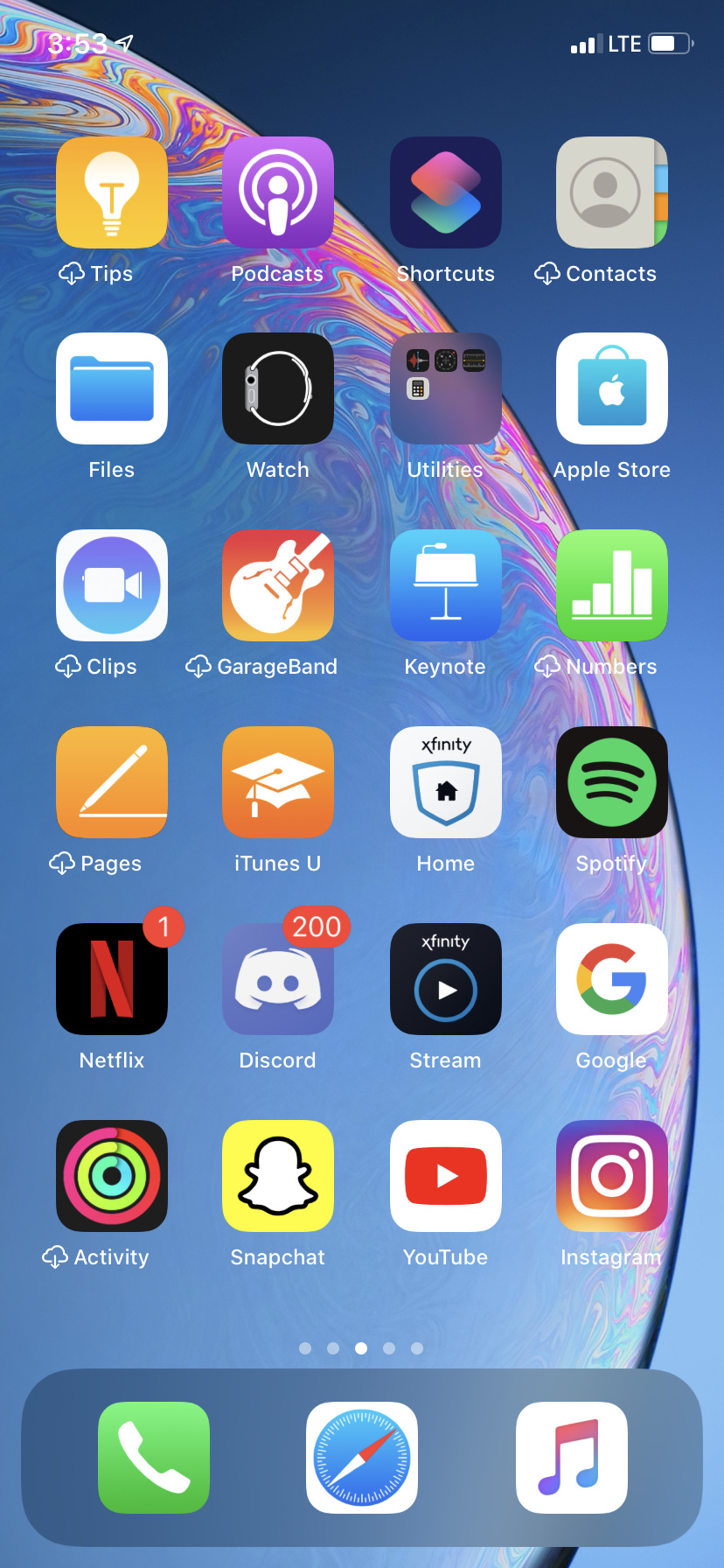The image is a screenshot of a smartphone home screen taken at 3:53, featuring a blue background adorned with a close-up of a water drop displaying an iridescent, oil-slick-like design. The status indicators reveal three out of four signal bars and a battery with three-quarters remaining. The home screen is organized into six rows, each containing four app icons with their respective names below. The apps displayed, from top left to bottom right, include: Tips, Podcasts, Shortcuts, Contacts, Files, Watch, Utilities, Apple Store, Clips, GarageBand, Keynote, Numbers, Pages, iTunes U, Home, Spotify, Netflix, Discord, Stream, Google, Activity, Snapchat, YouTube, and Instagram.